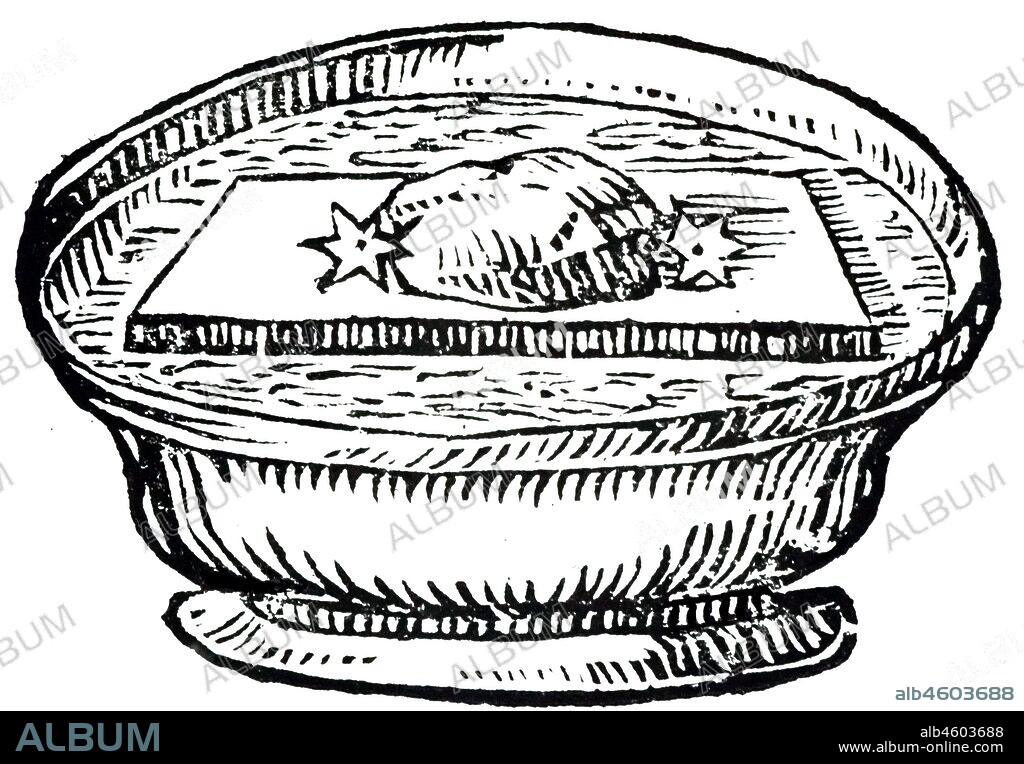The image depicts a detailed digital drawing featuring a round bowl set against a white background. Inside the bowl is a rectangular board, atop which rests an object resembling a rock or possibly a round loaf of bread. Flanking this object are two stars, adding a celestial touch to the scene. The bowl appears to be filled with water. The drawing, executed in black against white, subtly emulates pencil art but is digitally rendered. A recurring grey watermark reading "ALBUM" overlays the entire image. At the bottom of the image, a black horizontal strip contains text. On the left side of this strip, in blue or grey lettering, the word "ALBUM" is displayed. On the right side, the code "ALB4603688" and the URL "www.album-online.com" are printed in white. Above this banner, the code "ALB4603688" is also visible in a distinct greeny-grey color.